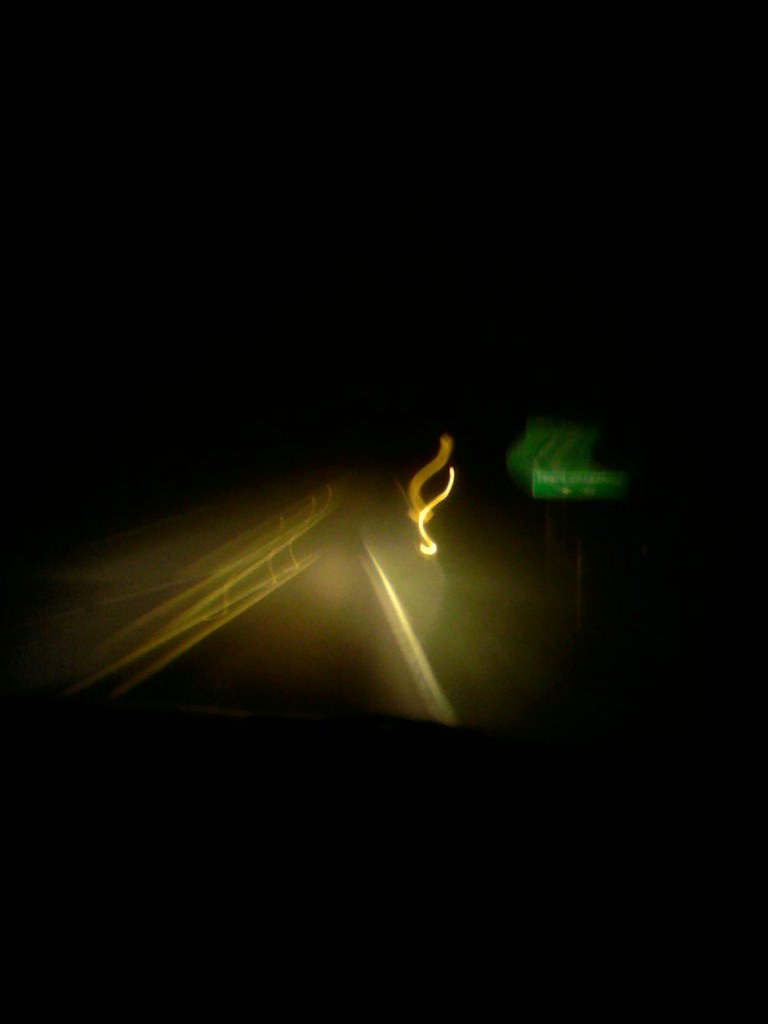This photograph, taken at night on a roadway, features a very dark and blurred composition. In the center left, the road stretches off into the distance, forming a triangular shape against the black background. The sides of the road are lined with yellow streaks of light, suggesting the photographer was moving while capturing the shot. To the right, two yellow curved lines of light ascend toward the top, possibly representing headlights. A rectangular green highway sign, located at the far right center, displays white text, though it is quite blurred. The sign appears to have wavy green patterns behind it, perhaps due to double exposure or motion blur. The overall scene is very dark, making it challenging to discern further details, but the interplay of yellow and green lights creates an intriguing and slightly surreal atmosphere.